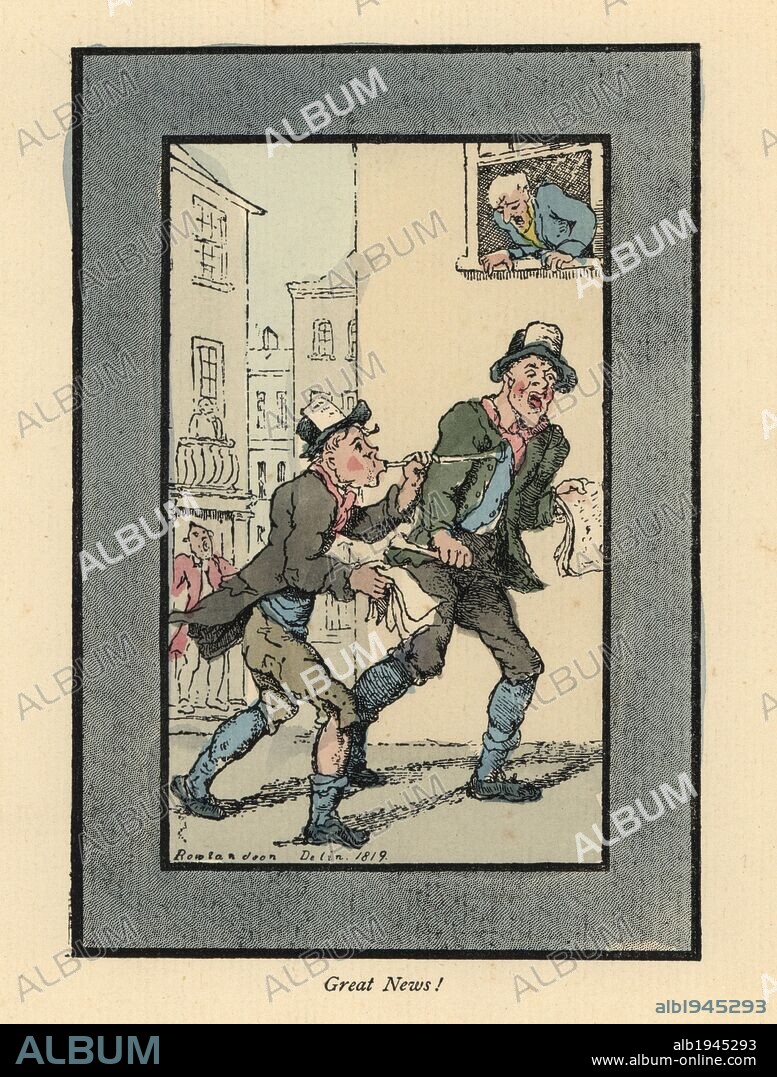The image is a detailed and intricately bordered cartoon illustration, possibly originating from around 1819, featuring a city street scene. The artwork is framed by a solid beige border and a series of thin black lines with gray spaces in between, creating a distinct visual separation. In the center, two somewhat disheveled men are depicted; one smaller figure annoys the taller one by blowing a horn. Both characters are similarly clad in green jackets, tattered pants, blue socks, and hats with small unreadable signs. Adding to the old-world city atmosphere, there's a man leaning out of a window in the background, and a variety of people are visible among the old buildings. At the bottom of the image, bold text exclaims, "Great News."